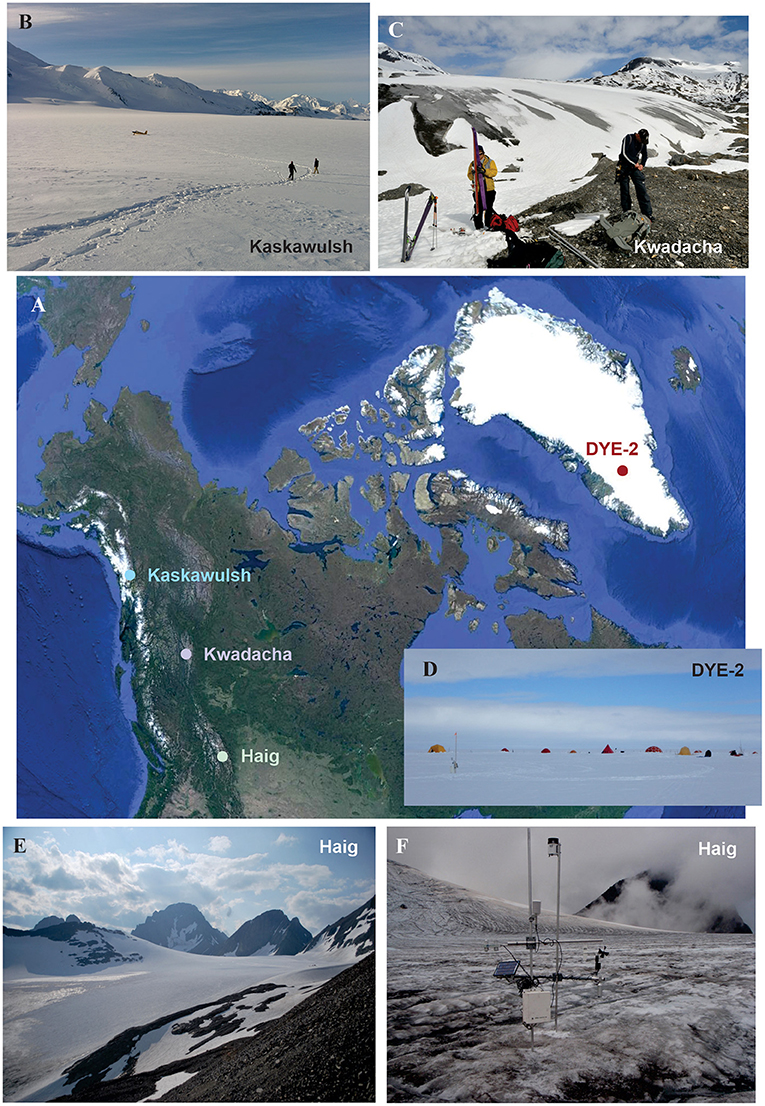The image is a vertical rectangle collage composed of several smaller rectangles showcasing different snow-covered locations. The two top horizontal rectangles feature snowy landscapes: the left one shows a pristine snow-covered field with hills in the background and two skiers under a clear blue sky labeled "Kaskawulsh," while the right one depicts a partially thawing snow-covered hill with exposed black and gray dirt, also showing two people preparing to ski, and labeled "Kwadacha." The central vertical rectangle is a detailed map illustrating parts of Canada and Greenland surrounded by dark blue water, with labeled regions such as "Kaskawulsh," "Kwadacha," "Haig," and "DYE-2." The bottom two horizontal rectangles, both labeled "Haig," depict contrasting scenes: the left one showcases a smooth snow-covered hill with prominent dark gray and black ridges under a cloudy blue sky, while the right one features a field with patchy snow and visible black dirt, obscured in the background by what appears to be white fog or smoke.